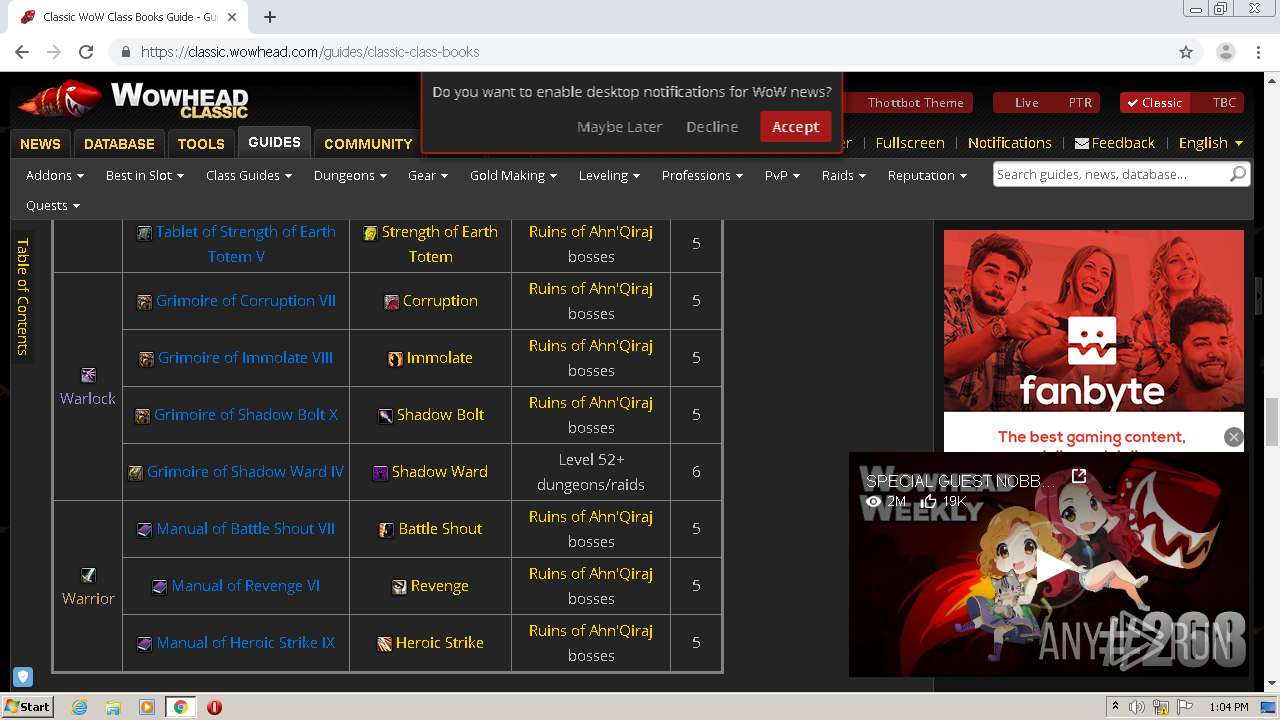This computer screen captures a horizontal rectangular image with multiple visual elements and text. At the top left corner of the screen, inside a black horizontal rectangle, is a logo featuring a red, shark-like figure with an open mouth and sharp teeth. To the right of this logo, in white capital letters, is "WOWHEAD," with the smaller yellow capital letters "CLASSIC" aligned directly underneath "HEAD." 

Centering the top edge of the black area is a red-bordered pop-up notification with a black background, asking, "Do you want to enable desktop notifications for WOW NEWS?" Below this query, there are options to either "Maybe later" or "Decline," but the "Accept" option is highlighted in white text inside a solid red rectangle.

On the left portion of the screen is a navigation menu with options in yellow and white capital letters. The sections listed are:
- NEWS (yellow)
- DATABASE (yellow)
- TOOLS (yellow)
- GUIDES (white)
- COMMUNITY (yellow)

To the left edge of the screen, there is a partially visible "TABLE OF CONTENTS" heading. Beneath it, columns of information are displayed, though some text is cut off or unclear. The first column lists "WARLOCK" and "WARRIOR." The second column, in blue font, includes "TABLET OF STRENGTH OF EARTH TOTEM 5." Further down this column and the others are items like "MANUAL OF BATTLE SNOUT" and other text too blurred to discern.

Along the right side of the screen, there are various advertisements, but specific details about these ads are not visible. The overall impression is of a dense and text-heavy interface, typical of a gaming or information website.